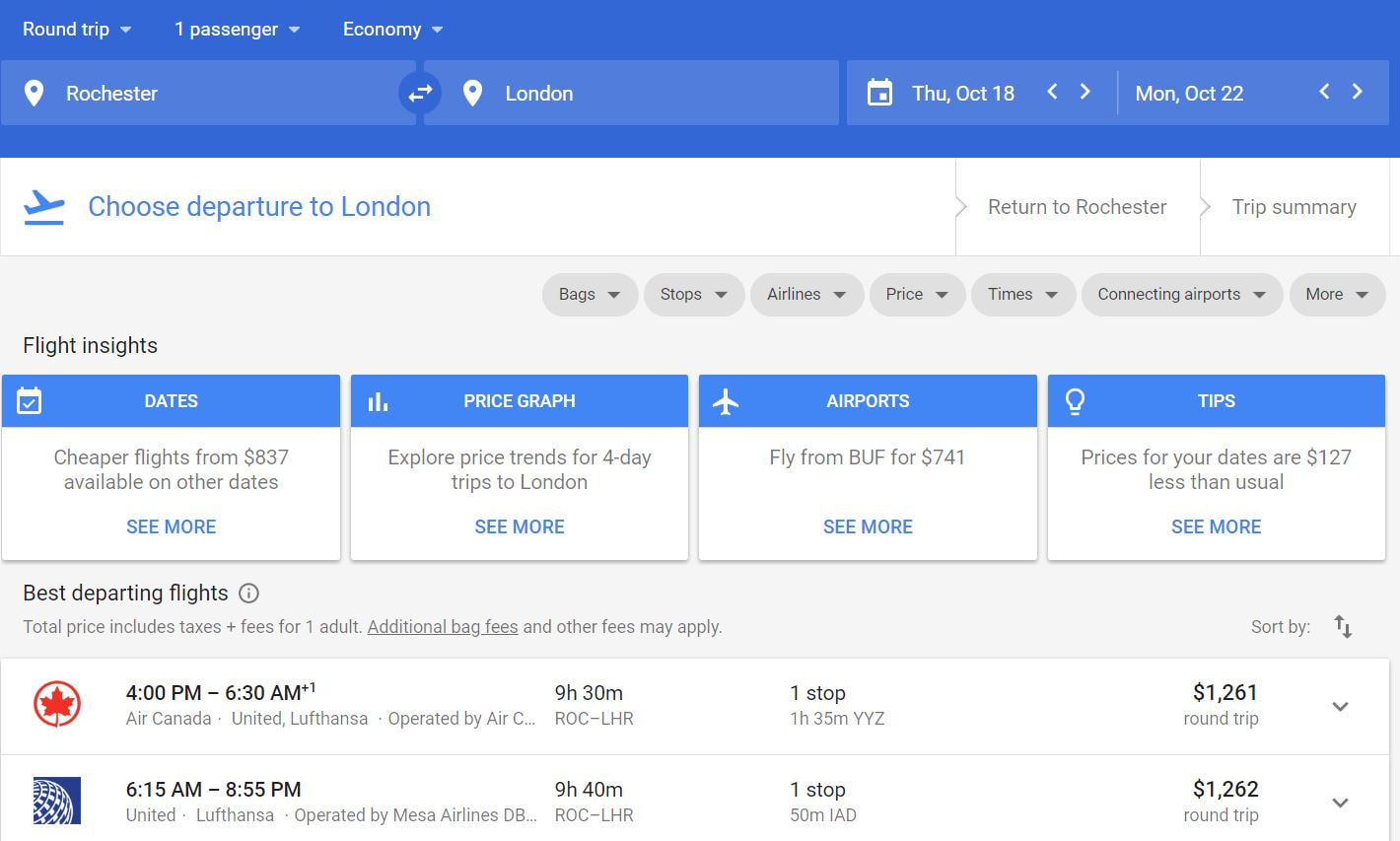Screenshot from Google Flights showing options for booking flights from Rochester to London. The search is for a trip departing on Thursday, October 18, and returning on Monday, October 22. The interface features Google's signature blue tabs, and displays various travel details:

- The "Choose Departure" and "Return to Rochester" options are visible, along with a trip summary.
- Flight insights indicate that there are cheaper flights available on other dates.
- A price graph provides an overview of price trends.
- The cheapest available flights from Buffalo (BUF) start at $741.
- A tip indicates that the prices for the selected dates are $127 less than usual.

Two prominent flight options are listed:
1. **Air Canada**:
   - Departure: 4:00 PM
   - Arrival: 6:30 AM (next day)
   - Duration: 9 hours 30 minutes
   - One stop: 1 hour 35 minutes
   - Total price: $1,261 (including taxes and fees; additional bag fees may apply)
   - This is a round trip.

2. **United Airlines**:
   - Departure: 6:15 AM
   - Arrival: 8:55 PM
   - Duration: 9 hours 40 minutes
   - One stop: 50 minutes
   - Total price: $1,262 (including taxes and fees; additional bag fees may apply)
   - This is a round trip.

The screenshot highlights the comprehensive details provided by Google Flights for travelers seeking to plan their trips efficiently.